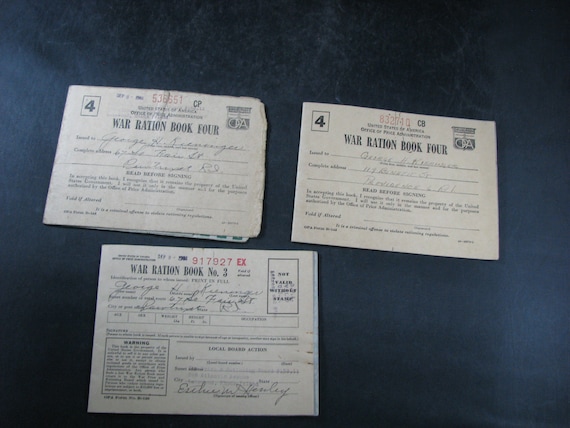The photograph showcases three war ration books from the United States, set against a blue background. The top two books, both titled "War Ration Book 4," feature identification numbers "536651" on the left and "83274Q" on the right. Each of these books has a distinct shield logo on the upper right and the number "4" prominently displayed in a box on the upper left. Below them, the third booklet, titled "War Ration Book 3," bears the identification number "911917927." This book includes a small chart and a boxed warning about validity and stamps. Signatures are visible on all three ration books, with the name "George H" discernible, although the last name is unclear. Each card also prompts the individual to fill out their complete address, accompanied by the phrases "Read before signing" and "Void if altered."